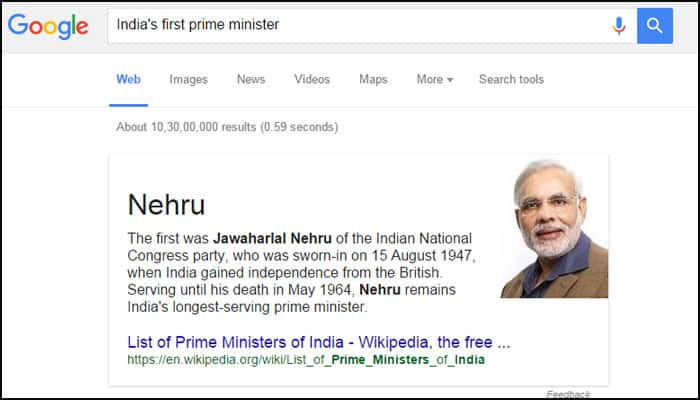The image shows a screenshot of Google's search engine interface. In the top left corner, Google's iconic logo is displayed prominently. Below the logo, there is a search box where the user has typed "India's first Prime Minister." To the right of the search box is a microphone icon, indicating the option to perform voice searches. Adjacent to the microphone is a blue magnifying glass button, which is used to initiate the search.

Beneath the search box are several tabs including "Web," "Images," "News," "Videos," "Maps," "More," and "Search tools." The results shown are currently under the "Web" tab. A fine print just below the tabs indicates that there are about "10,030,000,000 results" for this search query.

The primary search result is about Jawaharlal Nehru, identified as India's first Prime Minister. The text explains, "The first was Jawaharlal Nehru of the Indian National Congress Party who was sworn in on 15 August 1947 when India gained independence from the British, serving until his death in May 1964. Nehru remains India's longest-serving Prime Minister." A link to a list of Prime Ministers of India on Wikipedia is included at the end of the result description.